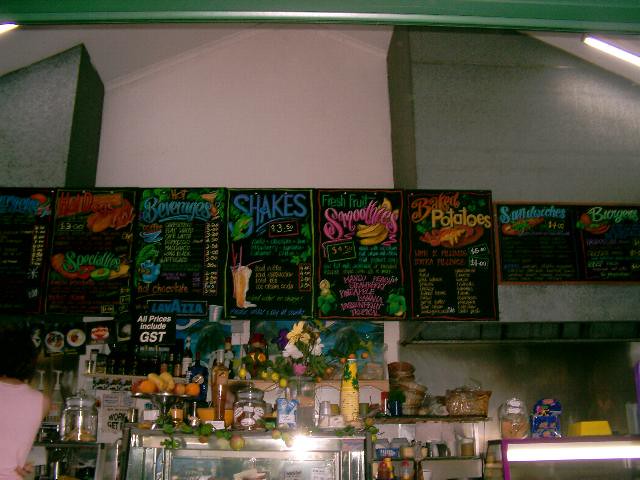The image captures the vibrant atmosphere of a smoothie and shake restaurant, immediately drawing attention with its colorful and dynamic menu displayed behind the register. The menu is an array of hues including blue, light green, darker green, pink, dark pink, yellow, and turquoise, adorned with large, elegant yet easily readable lettering. Sections on the menu clearly delineate the variety of offerings available, including beverages, shakes, potatoes, sandwiches, burgers, and more.

The counter is bustling with fresh, inviting elements—a fruit platter prominently shows off oranges, bananas, and apples, signaling the fresh ingredients used in the establishment's offerings. Behind the counter, a display case likely houses health-conscious milk options such as soy and almond milk. Clear containers line another section of the counter, which features a captivating light with a purple trim. Additionally, a yellow box adds a pop of color to the counter space.

On the counter adjacent to the fruit platter, there's a glass jar with a tan item inside, reflecting the overhead lighting and adding to the restaurant's lively and welcoming ambiance.